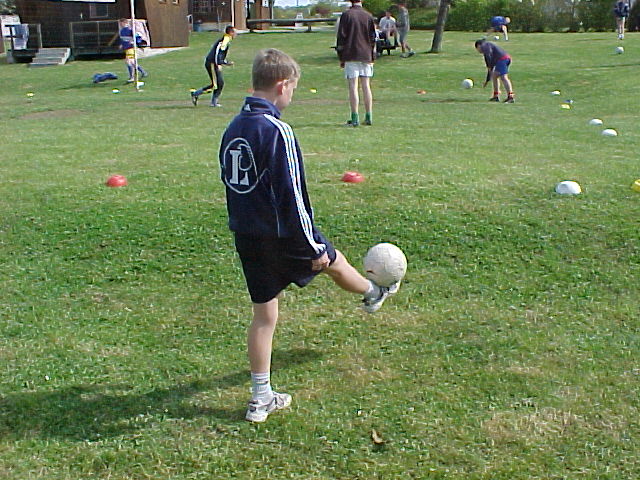In this detailed color photograph taken on a bright and sunny day, a young boy, approximately 10 to 12 years old with short blonde hair, is prominently featured in the foreground of a grassy field, possibly a park. The grass is lush, green, and neatly trimmed. The boy is wearing a navy tracksuit consisting of navy shorts and a navy jacket with white stripes running down the sleeves. He also sports white ankle socks and blue-and-white tennis shoes. He is skillfully balancing an all-white soccer ball on his right foot, suggesting he might be about to kick or lift it. 

Surrounding him, several other children and a couple of adults are also engaged in playing soccer, none donning uniforms, indicating a casual, friendly match. The people in the background vary in attire, with some in shorts and others in pants. There are red and white soccer balls scattered across the field. To the left side of the image, a brick building with a set of concrete steps and a possibly truncated flagpole can be seen, adding to the park setting. Additionally, a picnic table with seated individuals hints at onlookers enjoying the game.